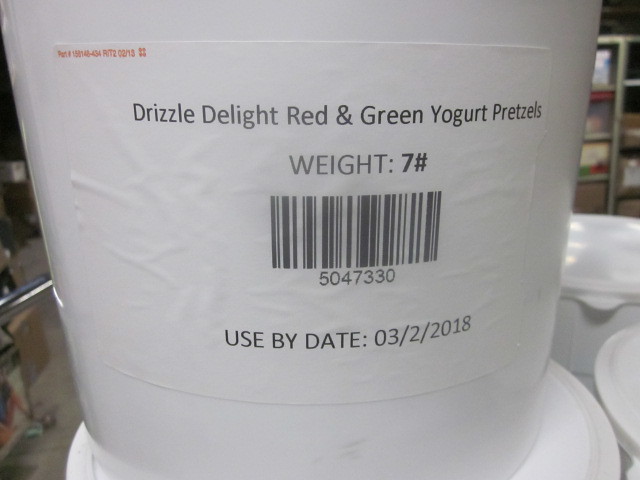This photograph features a large, round white container, resembling a bucket or barrel, prominently labeled "Drizzle Delight Red and Green Yogurt Pretzels." The label has black text and an additional red inscription that's not entirely legible. It includes the weight as "7 lbs," a UPC barcode, the number "5047330," and a "used by date" of "03/02/2018." The container occupies most of the frame and is stacked atop another identical container. To the right, several more similar white tubs are partially visible. The background reveals elements of silver shelving, poles, and possibly other items stored on shelves, suggesting the setting is likely a warehouse or the backroom of a store. On the left side, the warehouse floor can be seen along with a box and other miscellaneous items.